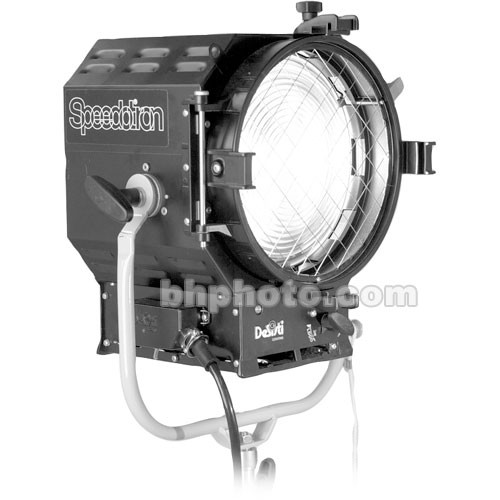The black and white image showcases a large studio spotlight, commonly utilized in stage or film production, mounted on a lighter stand for stability. The robust light source, identified as a Speedotron by the text on its side, features a Fresnel lens framed by adjustment knobs positioned at the 12, 3, 6, and 9 o'clock locations, allowing for precise directional control. The light is further equipped with a grate over the front to diffuse the beam, and a wire extending from its bottom runs out of the frame, indicating electrical connectivity. Notably, the light's body is housed in a U-shaped, metal-colored bracket that permits rotational mobility through T-shaped clamp screws on either side. Below the primary Speedotron branding, there are additional inscriptions suggestive of partnerships or secondary brands, including partially obscured text and a CBS sticker, hinting at its use in professional broadcasting. Moreover, a prominent watermark across the image reads 'bhphoto.com,' signifying the light's association with this retailer or source.